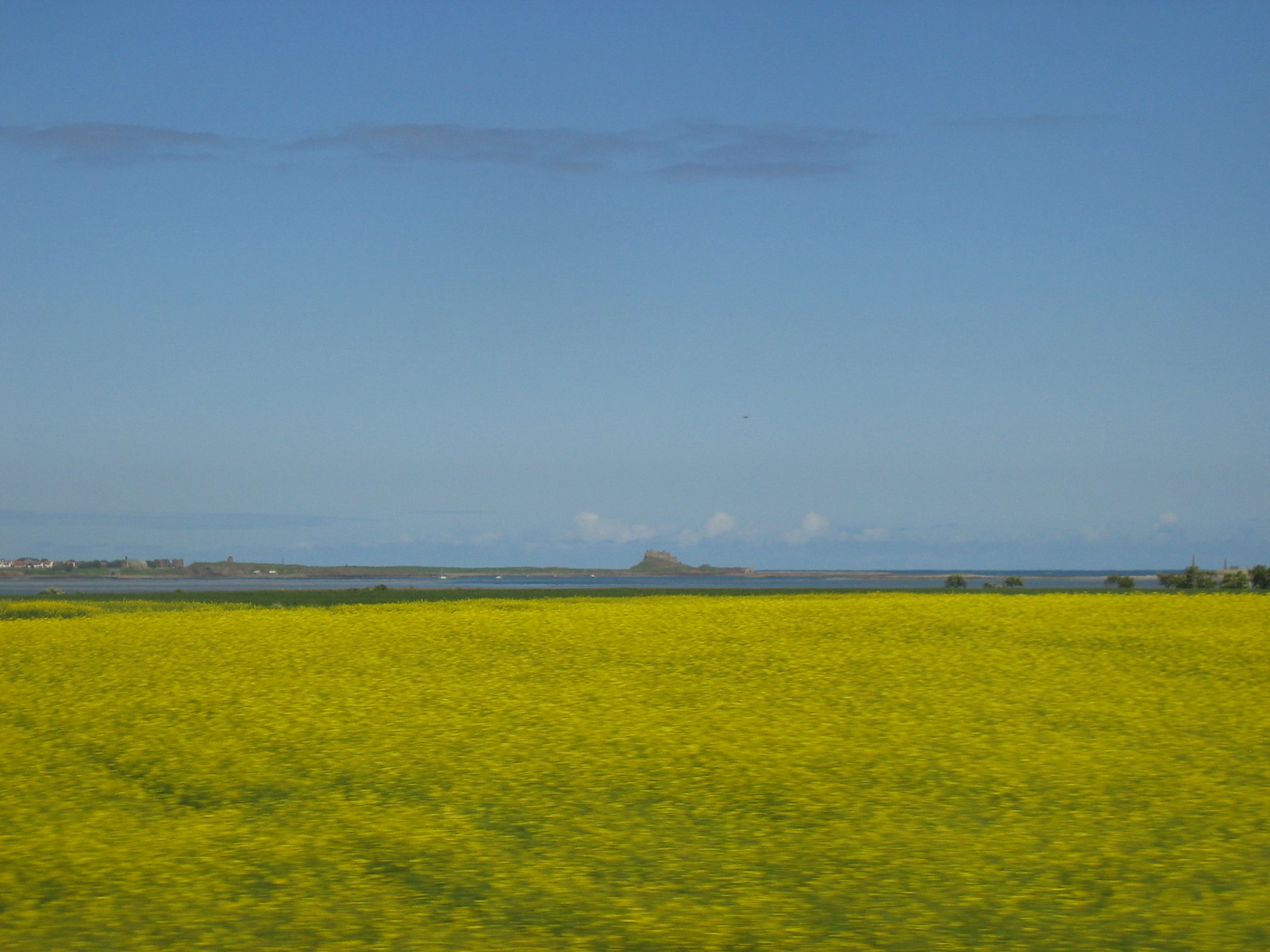The photograph captures a serene landscape with a rich blend of elements. At the forefront lies a flat field, mostly blanketed in vibrant yellow flowers interspersed with patches of green. Scattered within the field, particularly on the right side, are a few sparse trees boasting light green leaves. Beyond this, a large, blue-hued body of water stretches across the mid-ground, reflecting the daylight. Bordering the water on the left is a small, rural-looking town with sparse buildings, adding a touch of habitation to the otherwise natural scene. In the distance, majestically centered, a sizeable mountain or plateau rises, shrouded in a subtle haze that blurs its full definition and adds depth to the photograph. Above, the expansive sky transitions from a marine blue at the top, interspersed with a few elongated dark gray clouds, to a lighter blue closer to the horizon, portraying a typical daytime setting.